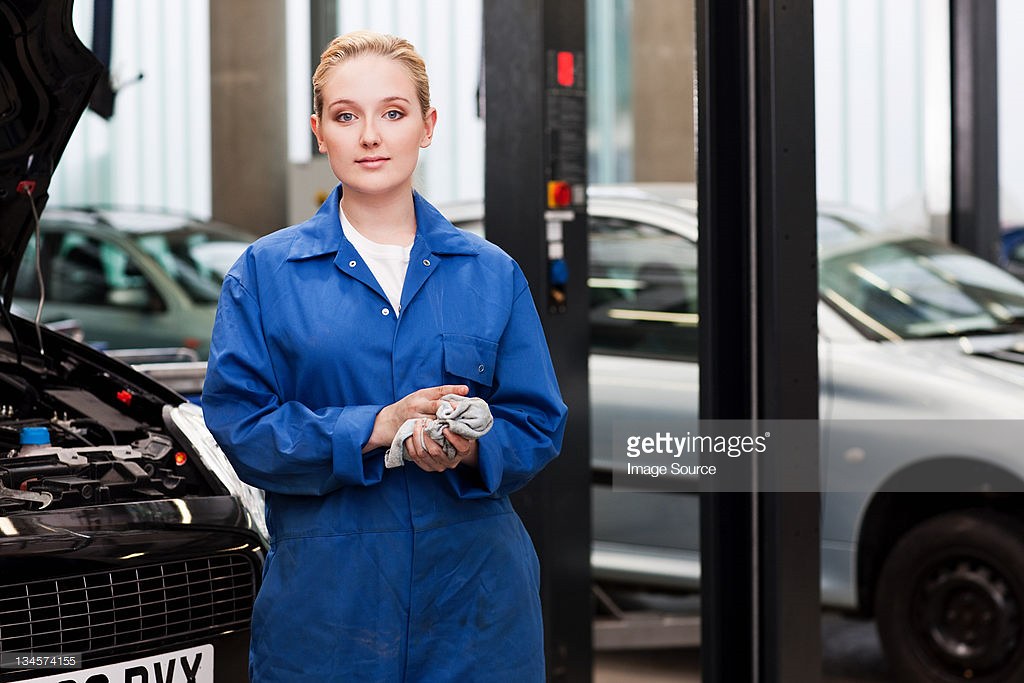The image captures a blonde, Caucasian female mechanic in a brightly lit, large mechanic shop. She is dressed in a vibrant blue jumpsuit with a white shirt underneath and has her blonde hair pulled back, possibly wearing makeup. She stands in front of a black sedan with its hood open, indicating she was recently working on the engine. Her hands, covered in grease or oil, are being wiped clean with a white rag that also shows signs of grease. The background features several sedans, including a silver one and a greenish one, near car lifts with buttons. The environment is filled with square-shaped, metal poles that are part of a car lift system. In the middle of the image, there is white text that reads "Getty Images, Image Source."